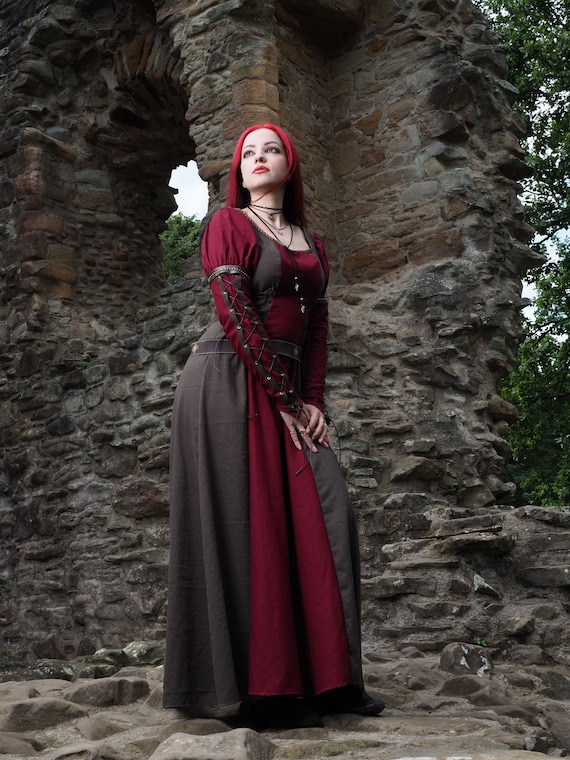The photograph captures a detailed image of a woman dressed in an elaborate medieval costume standing amidst the ruins of a crumbling castle. Her attire is a striking dress with brown panels on the sides and dark red segments in the center and on the long sleeves that extend beyond her wrists. Wrapped around her arm is a brown leather lace harness, adding to the intricate details of her outfit. She wears multiple black necklaces and a choker around her neck. 

Her hair, dyed red in the front and black at the back, cascades to just past her shoulders. She stands with one knee slightly bent upward, both hands resting on her upper thigh. Her expression is solemn, with dark lips enhancing her intense gaze. On her feet, she dons dark leather shoes that complement her medieval ensemble. The backdrop features a partially crumbled stone wall with a window, offering a glimpse of the sky through its upper section. Visible tree branches add to the mystique, further framed by the blend of gray and brown stone remnants of the ancient structure, creating a captivating and atmospheric scene.